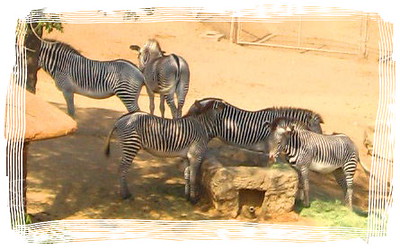This photograph captures a small group of five zebras within what appears to be a zoo enclosure. The edges of the image are uniquely bordered with wavy white lines, almost resembling strips of see-through tape. The scene is set on a light tan dirt ground, possibly desert-like, with a small patch of green grass in the bottom right corner. Two of the zebras, likely older, are walking away towards the top left of the image, distancing themselves from the remaining three younger ones who stand closer to the front. These three zebras are gathered around a makeshift feeding bowl, seemingly made from light brown stone or earth. One of the smaller zebras has their head dipped into this bowl, possibly eating. The zebras exhibit typical black and white stripes, although the lighting gives two of them a slightly lighter, almost grayish appearance. There's also shade cast over them, suggesting they are under a tree. A small white fence can be faintly seen in the background, adding to the enclosure feel. The overall photograph isn't particularly sharp, lending it an impressionistic quality.